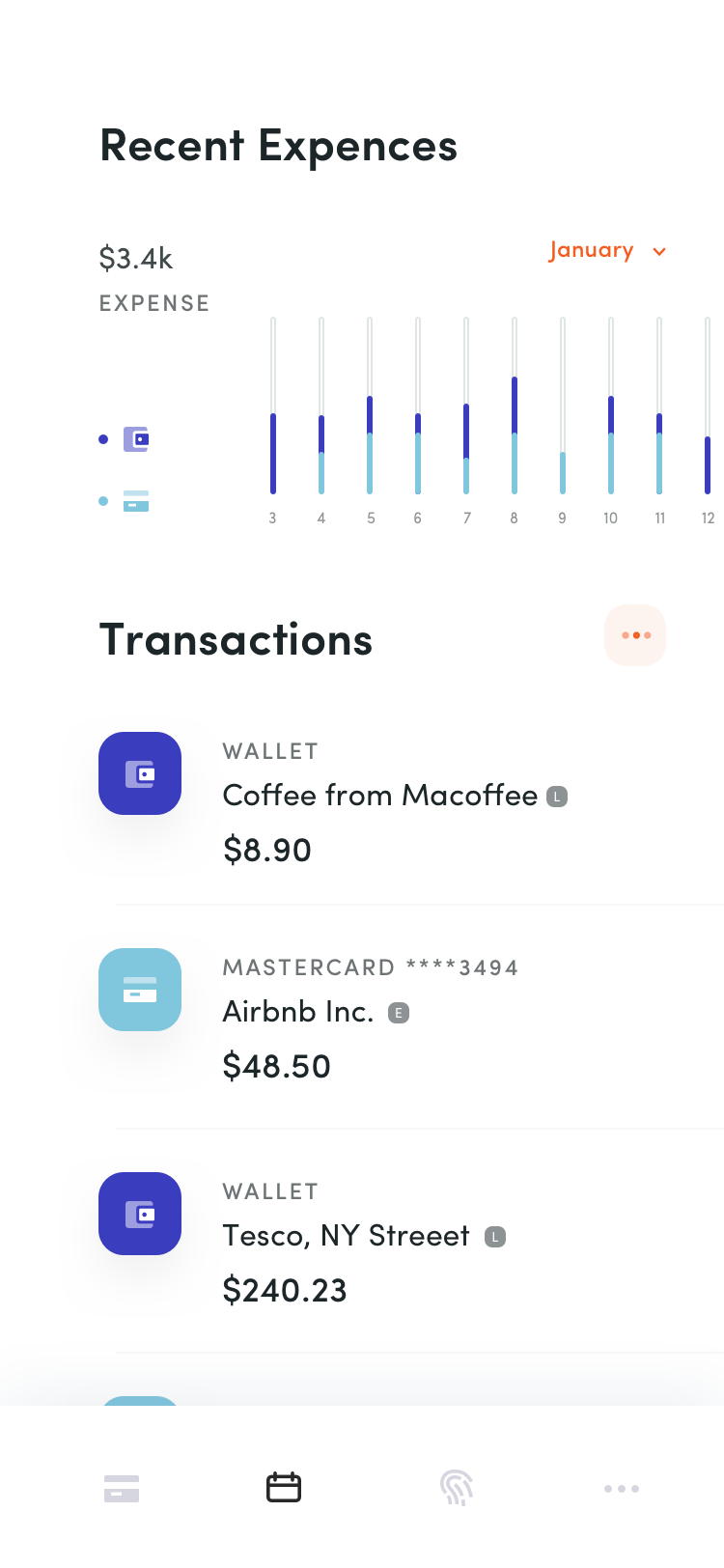This image is a detailed screenshot from a smartphone app displaying recent expenses against a white background. At the top, in black font, it reads "Recent Expenses." Below this header, on the left side, the figure "$3.4K" is prominently displayed. Underneath this figure, in small, purple, capitalized letters, it says "EXPENSE."

To the right, in red text, the word "January" is seen, accompanied by an inverted outline that resembles a triangle, indicating a drop-down menu. The central portion of the image features a bar graph with two colors: purple and light blue. Although the legend for these colors is absent, it can be inferred that purple represents "Wallet" transactions and light blue represents "MasterCard" transactions.

Below the bar graph, under the headline "Transactions," there is a list of three recent transactions. The first transaction is marked by a purple square with rounded corners, labeled "Wallet." It details a purchase of coffee from McCaffey costing $8.90. 

The second transaction is identified with a blue square with rounded edges, matching the blue in the bar graph. It is labeled "MasterCard" and specifies the last four digits of the card. This entry shows a payment to Airbnb Inc. amounting to $48.50.

The final transaction on the list is again marked by a purple square, labeled "Wallet," detailing a purchase from Tesco NY Street for $240.23.